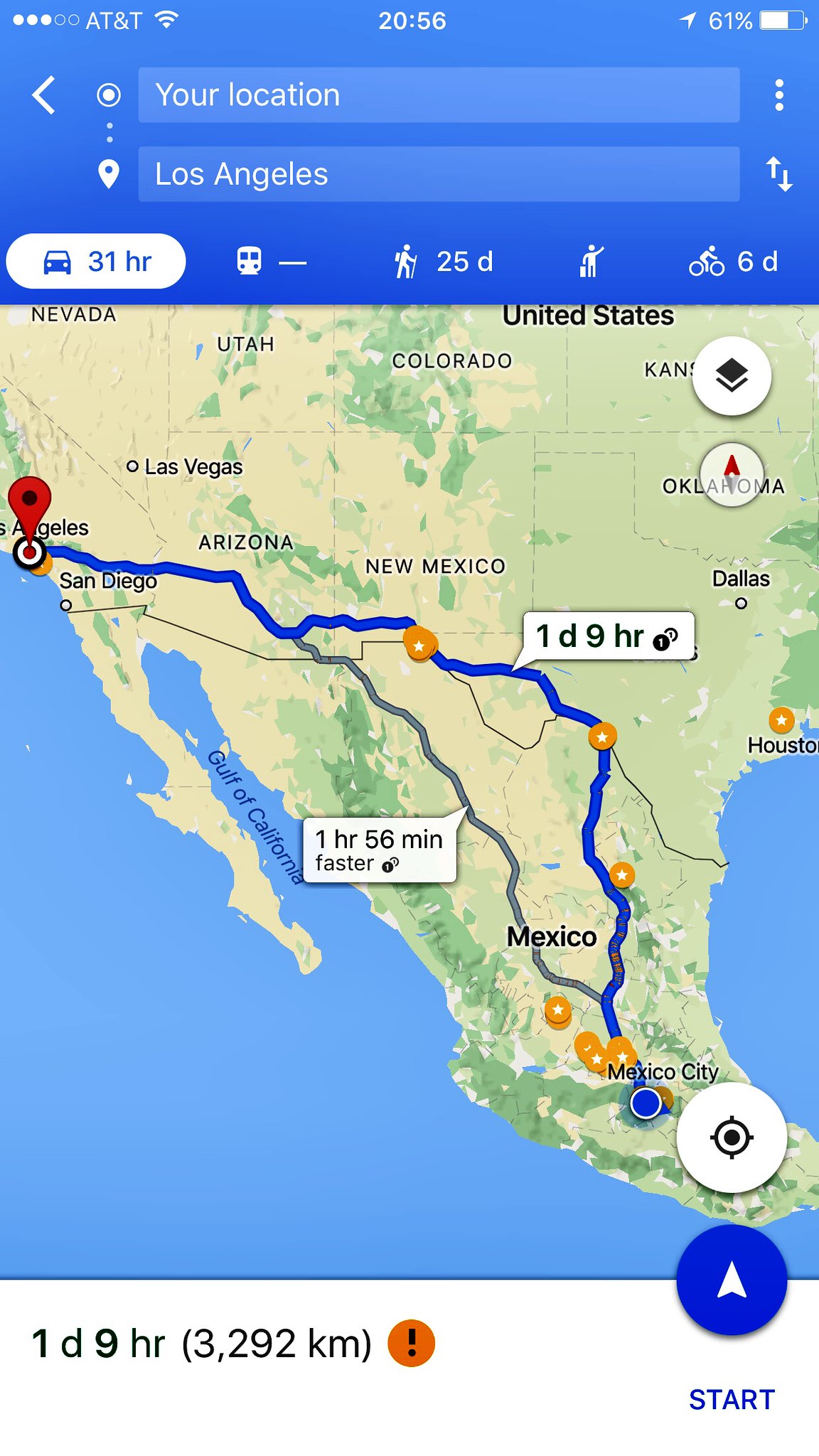The image depicts a smartphone screen displaying a navigation app with driving directions from Mexico City to Los Angeles. At the top of the screen, the standard status bar indicates the phone is on AT&T's network, shows a Wi-Fi symbol, signal strength, and the time, which is 8:56 PM. On the top-right corner, the battery indicator shows a 61% charge.

Below the status bar, a search field is pre-filled with 'Los Angeles' as the destination. Underneath, a blue driving icon is highlighted, indicating the selected mode of transportation. It shows an estimated travel time of 31 hours by car. Additional icons suggest alternative travel methods with corresponding times: a train (25 days), hiking (unrealistically marked as 25 days), and bicycling (6 days).

The main part of the screen displays a map of the southwestern United States, detailing a route from Mexico City to Los Angeles. Key states such as Nevada, Utah, Colorado, Kansas, Oklahoma, Arizona, New Mexico, California, and Texas are visible along with major cities including Las Vegas, San Diego, Los Angeles, Dallas, and Houston. Mexico City is marked at the starting point.

Two routes are indicated on the map. The primary route, represented by a thick blue line, estimates a travel time of 1 day and 9 hours (3,292 kilometers). An alternative, more direct route is noted to be 1 hour and 56 minutes faster. A red or orange circle with a black exclamation mark is placed at the bottom, possibly indicating a warning or advisory for the journey.